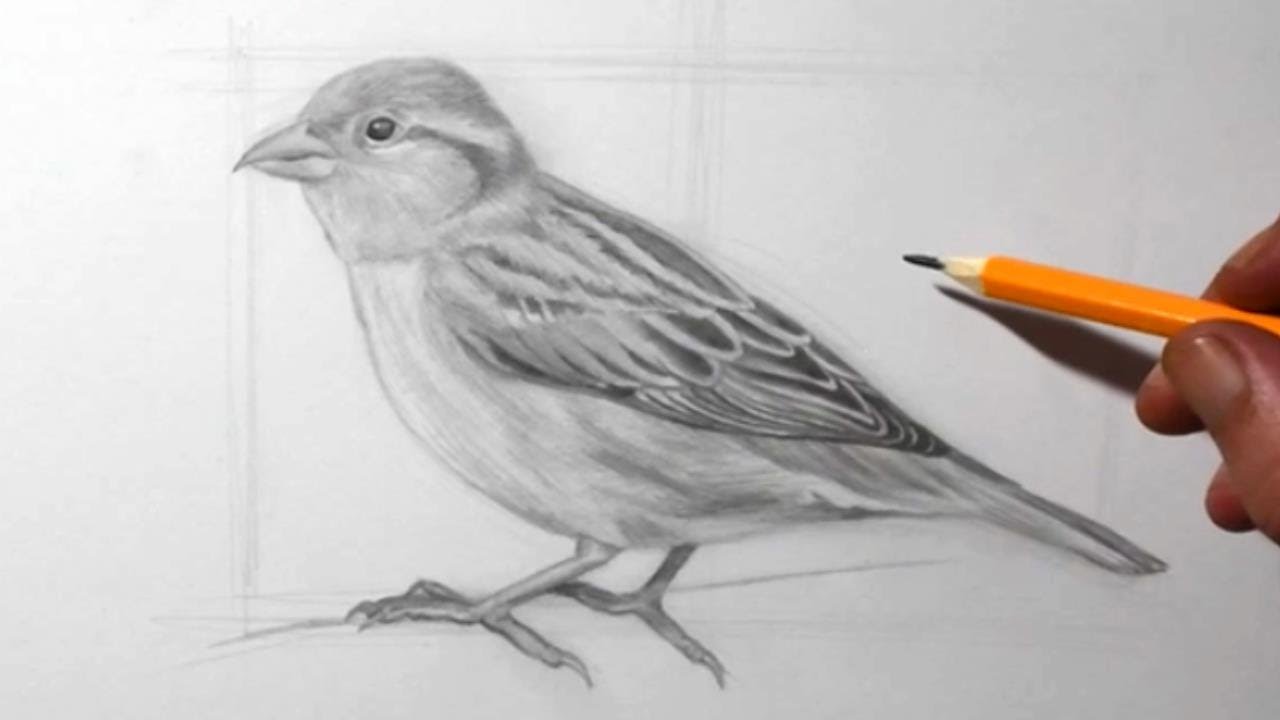The image depicts a detailed pencil sketch in grayscale of a small bird, which appears to be a sparrow, being drawn by an artist. The artist uses an orange pencil with a dark, likely charcoal lead. The artist's thumb, index finger, and another fingertip are visible, holding the pencil prominently. The bird is shown in a side profile, with one visible eye and a beak, perched with its feet on what seems to be an unfinished surface. Its feathers are intricately detailed, showcasing various shades of gray and white. In the background, there are square sections resembling window panes, each approximately the same size as the bird. While the bird itself appears nearly complete, portions of the background and perch remain unfinished. The overall scene is a black-and-white photograph capturing this work-in-progress.